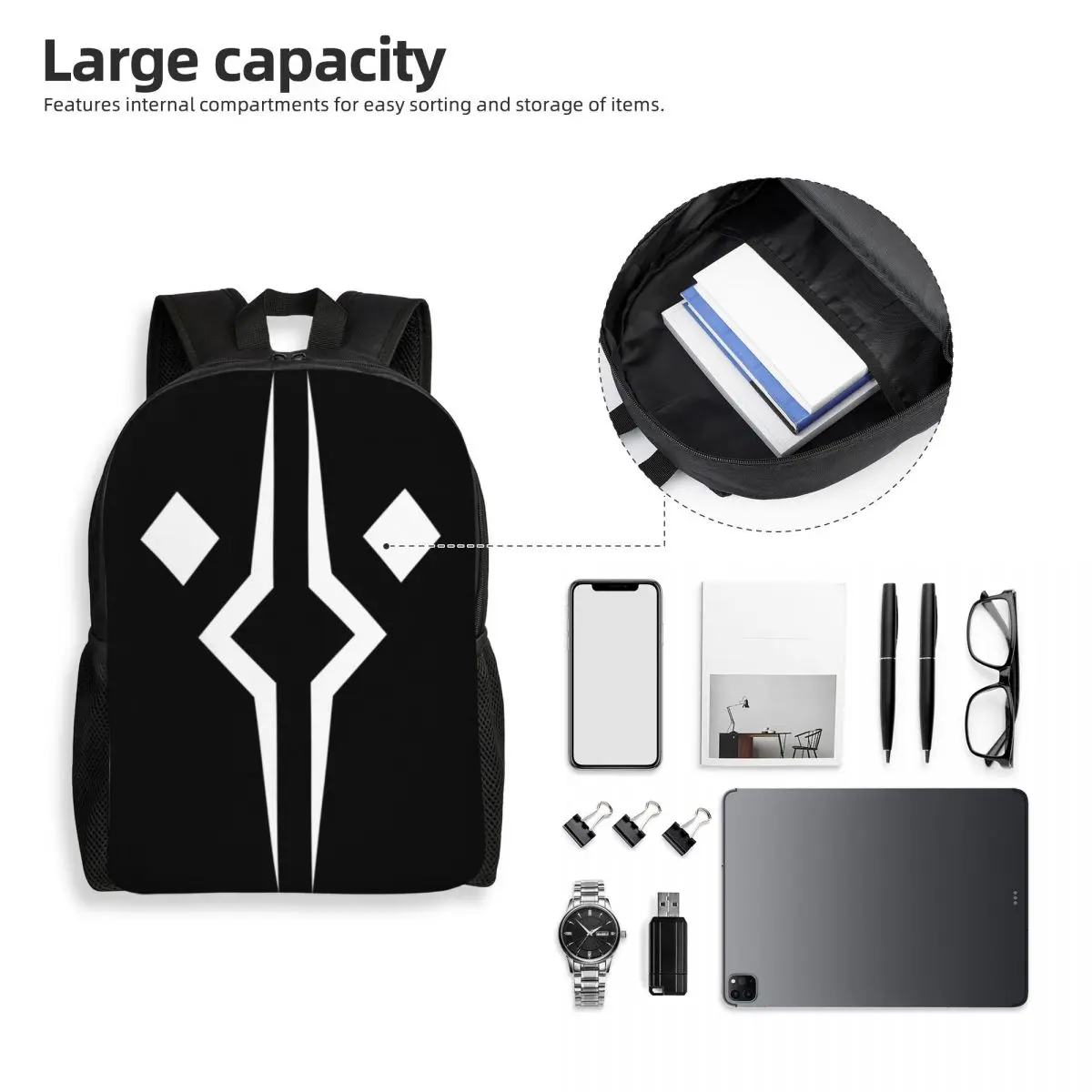This advertisement showcases a versatile black backpack with intricate white geometric designs, consisting of two vertical lines that mirror each other and two diamond shapes on either side. In the upper right corner, black lettering states "Large Capacity," emphasizing its internal compartments designed for easy sorting and storage. The left side of the image features the backpack, highlighting these compartments with an open flap revealing space suitable for books and other items. The right side of the advertisement illustrates the backpack's storage capacity by depicting items such as a phone, a notepad, pens, eyeglasses, paper clips, a watch, a USB drive, and a laptop. These visuals effectively convey the backpack’s utility for organizing and holding various everyday essentials.